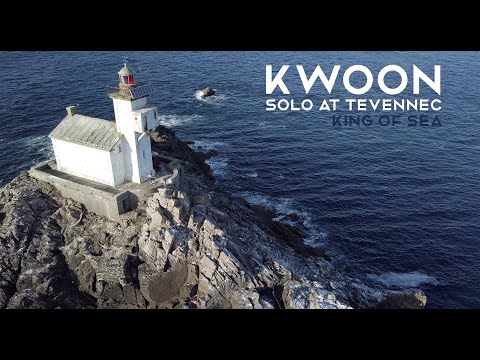This rectangular daytime photograph captures a striking lighthouse perched atop a large, rocky island in the ocean. The rocky formation, mostly gray and white, forms a natural base, extending from the lower left and sloping downward to the lower right of the image. Atop the rock, there's a substantial stone courtyard, fenced in and providing a sturdy foundation for the structures above. A white tower rises from the base, crowned with a lighthouse whose top is accentuated with red-painted windows. A veranda-like walkway encircles the lighthouse, offering panoramic views. Adjacent to the tower is a white building with a sloped gray roof and a chimney, serving as the living quarters. The background fades into the vast, blue sea, highlighting the solitude and prominence of the lighthouse. In bold white text in the upper right corner, the caption reads, “KWOON, Solo at Tevaneck,” with “King of the Sea” beneath in blue print.